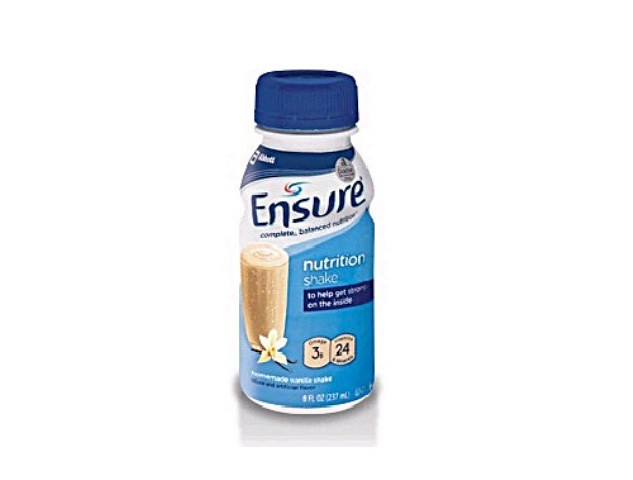The photograph showcases a plastic bottle of Ensure nutrition shake, displayed against a green screen, which gives it a uniformly vivid background. The image quality is somewhat lower resolution. The bottle prominently features the Ensure logo, which consists of dynamic swirls incorporating red and green hues, forming a circle that elongates at the top right and bottom left. The brand name is clearly spelled out as "ENSURE." This particular shake is the vanilla flavor, denoted by an image of a vanilla flower, and labeled "Vanillin" at the bottom. The bottle includes nutritional information and serving size details; it seems to be around 8 fluid ounces, judging by its proportion. Topped with a blue plastic cap, the entire bottle is made from easily disposable plastic.